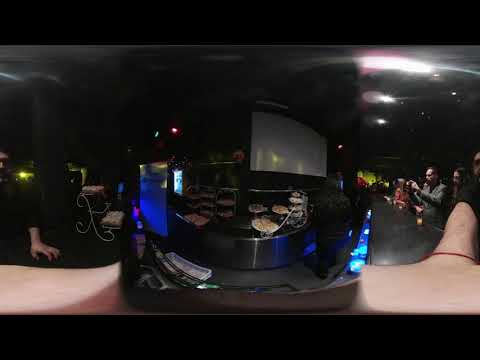The image depicts a dark, possibly distorted scene, resembling a photograph taken with a fisheye lens. In the center of the image, there appears to be a black square or cube showing an image that includes a long table filled with food items, possibly dishes on a grill or table. This central image is somewhat curved and seems to be situated on top of a white person's forearm, which extends across the bottom of the picture and includes a visible finger on the right. On both sides of this central cube, multiple people are standing or seated in what looks like a bar or restaurant setting. There's a blue glow under the bar and overhead white lighting, contrasting with the dark main color of the image. On the right side, several individuals appear to be waiting near a counter, while an individual in a black shirt is standing by some steps on the left. Additionally, a white movie screen is visible in the central image, adding to the complexity of the scene.